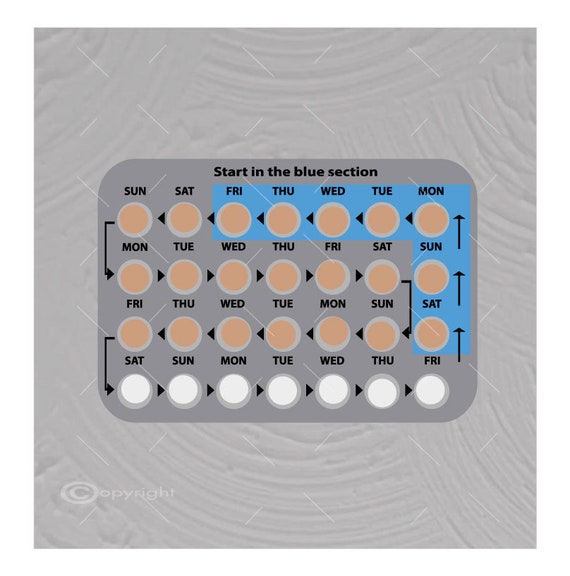The image depicts a detailed drawing of a birth control panel or contraceptive blister pack. The rectangular drawing, characterized by its rounded edges, shows a systematic layout designed to help users track their daily pill intake for a month. At the top of the panel, the text instructs to "start in the blue section," which begins on a Friday, indicated as "F-R-I" in the blue section. The subsequent arrow directs to Saturday, labeled "S-A-T," and then to Sunday, abbreviated "S-U-N." The days of the week continue sequentially in this manner across the top and snake down through the panel, changing direction at the end of each row to lead back the other way. Each day of the week is repeated across four weeks, with the first three weeks' pills colored pink and the final week, which is the placebo week, represented by white pills. These placebo pills are chemically inactive and align with the body's natural menstrual cycle. The blue section's color coding ends on Friday, after which the pills continue in a standardized layout. Additionally, the drawing features a watermark with cross-hatched lines and a copyright notice in the bottom left corner, indicating it may be a stock photo.